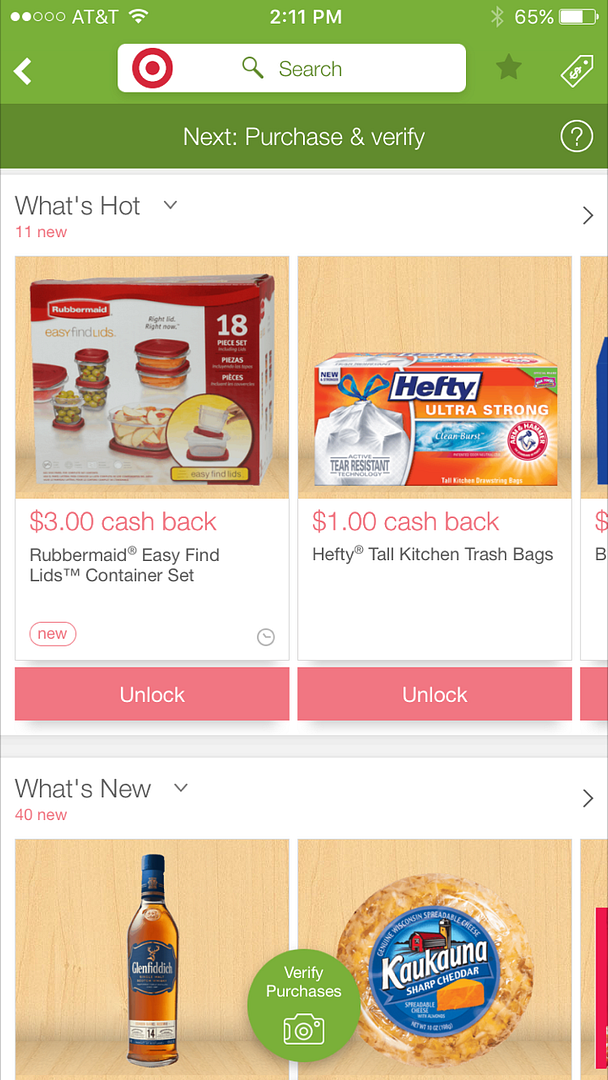This image is a detailed screenshot from the Target mobile shopping app, showcasing its green and white themed interface adorned with the recognizable red and white Target logo at the top center within a white search bar overlaying a green banner. Directly below is a darker green banner displaying the options "Next," "Purchase," and "Verify." The main section of the image features a horizontally scrollable list labeled "What's Hot, 11 new," with visually enticing product images. The first item displayed is a boxed set of Rubbermaid Easy Find Lids Container Sets tagged with a $3 cashback offer. Next to it is an orange Hefty Tall Kitchen Trash Bags box offering a $1 cashback. A partially visible item is adjacent to these products. Further down, the section labeled "What's New, 40 new" features a wheel of cheese and a bottle of alcohol, highlighting the app's diverse product range.